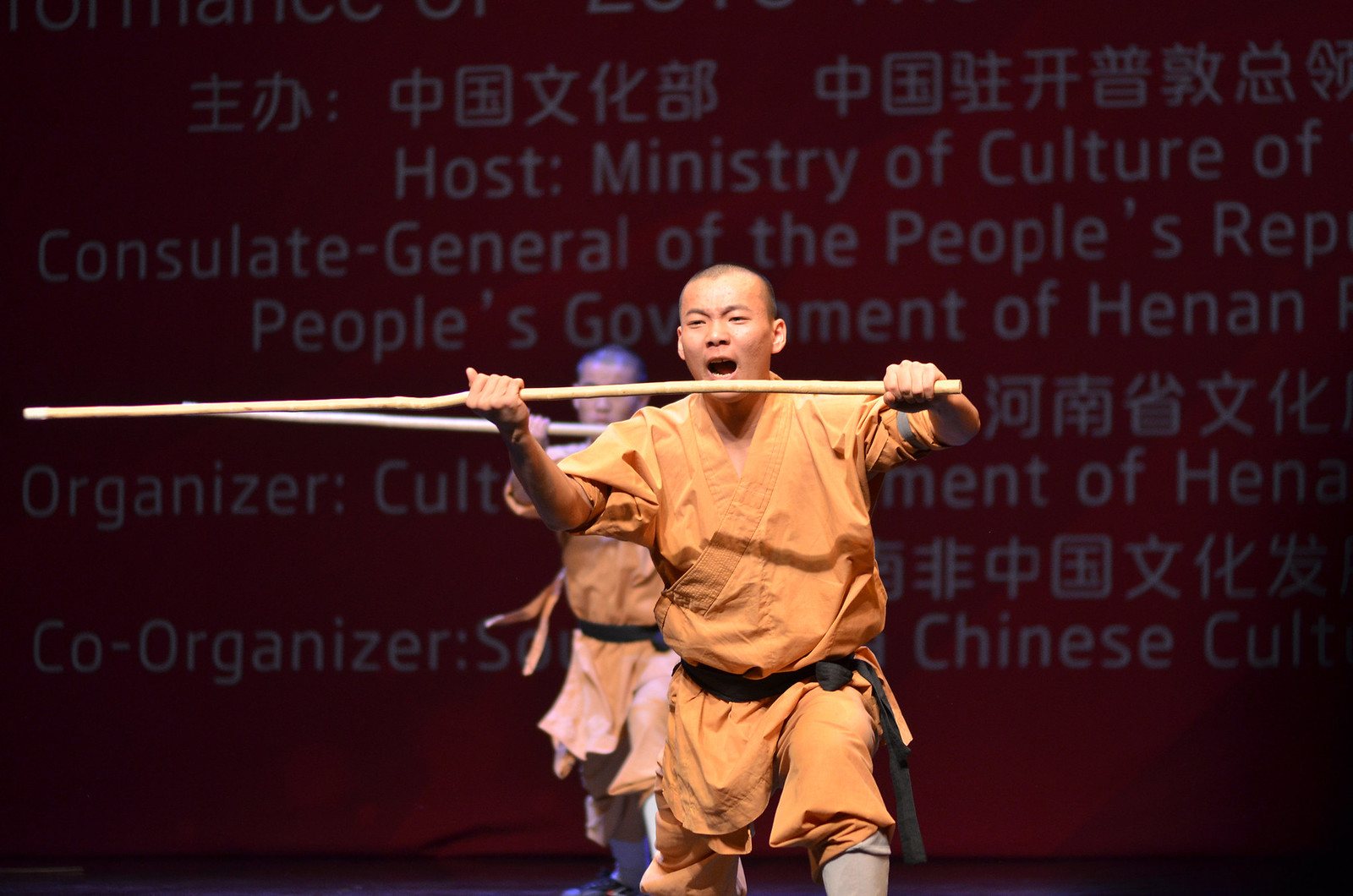In the image, we see a detailed and dynamic scene from a martial arts presentation, likely a competition or demonstration. At the forefront is a gentleman dressed in a light orange martial arts uniform with a black belt, holding a long, thin wooden stick. His posture is one of intensity as he lunges forward, mouth wide open in a shout, his brows furrowed in concentration. The spotlight sharply illuminates him, showcasing his almost bald head and the vivid expression of his face.

Behind him, another figure, similarly attired and wielding the same type of stick, is visible but blurred, emphasizing the motion and energy of the scene. Together, these martial artists appear to be executing a synchronized move.

In the background, there is a large red banner with white text, partially written in Asian characters and partially in English. The English text reads: "Host Ministry of Culture of... Consulate General of People's Republic, People's Government of Henan, Organizer and Co-Organizer, Chinese." Although the text is somewhat cut off, it's clear that the event is organized under significant cultural and governmental auspices. The darkened background with its spotlight effect and the prominent banner adds context and depth to the dramatic martial arts display happening on stage.